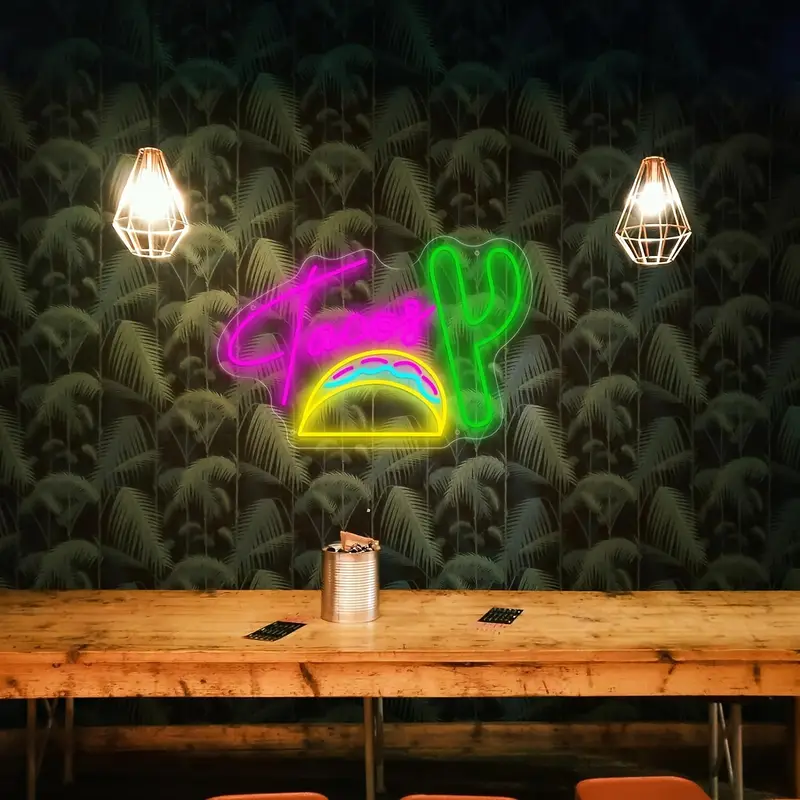This vibrant, detailed rendering captures the interior of a restaurant. Centered on the back wall is a neon sign in pink script reading "tacos," with a bright green cactus beside it. Below the word "tacos," a yellow hard shell taco contains colorful elements, including purple onion arcs and a blue wavy line. Framing this eye-catching neon sign are two hanging light fixtures with exposed bulbs. The background of the wall features green fronds set against a black backdrop, enhancing the lively atmosphere. In the foreground, there's a wooden counter with a silver can and some black menus on it. Red stools are partially visible, indicating seating arrangements.